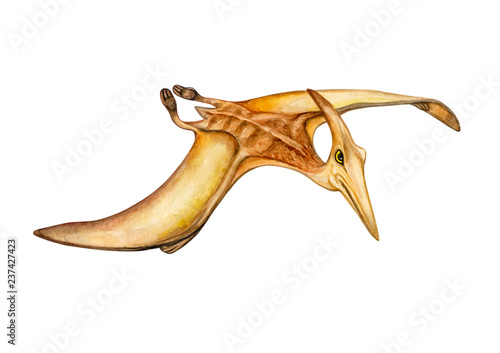The image is an animated portrayal of a flying pterodactyl, rendered in a hand-drawn style with watercolor shading. The pterodactyl, depicted in realistic detail, showcases various shades of brown with accents of black, yellow, orange, and amber, making it look lifelike rather than stylized. The background of the image is a minimalist white and gray, ensuring that the pterodactyl remains the central focus. It is captured in mid-flight with both wings fully extended; the wing closest to the viewer curves slightly upward and back, while the far wing curves downward. The pterodactyl's elongated beak and a head that tapers to a point further enhance its distinct features. Its eye is illustrated with a yellow iris and a black pupil, gazing to its right and slightly upward. Vertically positioned text on the side of the image reads, "Adobe stock," followed by the number "237-427-423" in parentheses. This image, likely intended for educational purposes, provides intricate details that could be used to teach about prehistoric creatures.